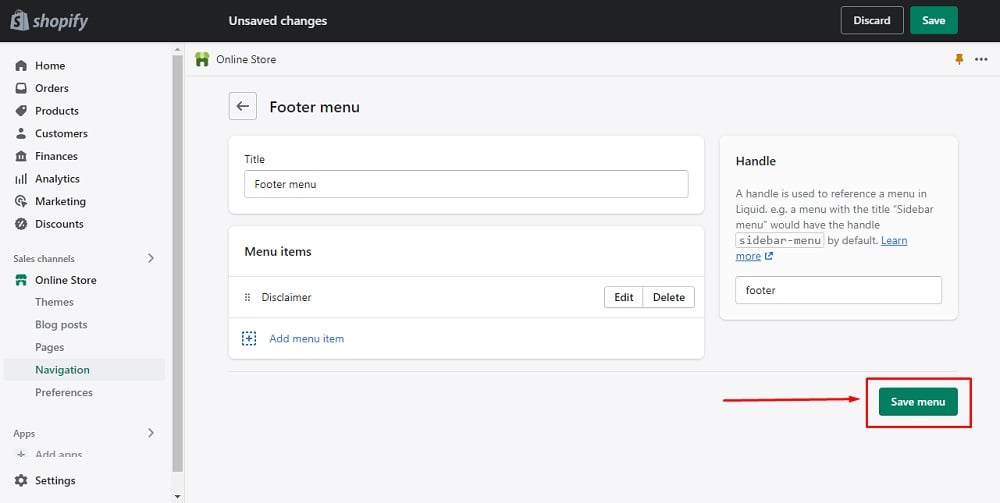**Screenshot of an Active Shopify Web Page**

In the image, a screenshot of a Shopify web page is displayed. The top left corner prominently features the "Shopify" logo set against a black navigation bar. Dominating the center of this bar is an alert-style text that reads "Unsaved changes," indicating that modifications have been made but not yet saved. On the far right side of the black bar, two buttons are visible: a black "Discard" button and a green "Save" button.

Beneath the black navigation bar, a sidebar menu on the left lists various navigational options: Home, Orders, Products, Customers, Finances, Analytics, Marketing, and Discounts. Additionally, there's a section labeled "Sales Channels," with the "Online Store" option currently highlighted. At the very bottom of this sidebar is a "Settings" button. Scrolling functionality is facilitated by a small scroll bar positioned to the right of the sidebar.

The main content area focuses on the "Online Store" settings, specifically the "Footer Menu." A back arrow is positioned next to the footer menu heading. Below, there's a "Title" field with an input box for customization. 

Further down, the "Menu Items" section appears, currently showing a single item, "Disclaimer." A plus symbol and the text "Add menu items" allow users to add more menu entries. To the right, a "Handle" section provides a description explaining how handles reference menus in Liquid, with an example for clarity. A blue "Learn more" link is also present for additional information.

In the bottom right corner of the main content area, a "Save menu" button is prominently displayed, indicating the option to save the current menu settings.